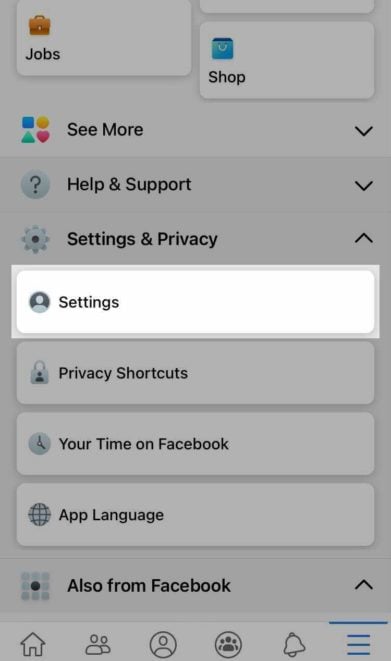This screenshot captures the settings menu of the Facebook mobile application. At the top of the screen, there is an orange briefcase icon adjacent to a "Jobs" section, followed by a blue handbag icon next to a "Shop" button. Below these options is a "See More" link, leading to additional features. The menu further includes "Help & Support," "Settings & Privacy," and the highlighted "Settings" section. 

Within the "Settings" subsection, users can manage "Privacy Shortcuts," review "Your Time on Facebook," select "App Language," and explore options "Also from Facebook." This screenshot appears to be user-captured to provide details about navigating to and viewing the various settings options on the Facebook mobile app.

At the bottom of the screen, the navigation bar includes a home icon, a profile icon (depicting two individuals), a user account icon, a groups icon (depicting three people), and a notification bell. The currently highlighted three-line or "hamburger" menu icon, leads to the displayed settings and privacy options. This detailed depiction illustrates how a user can access and modify their Facebook mobile settings.